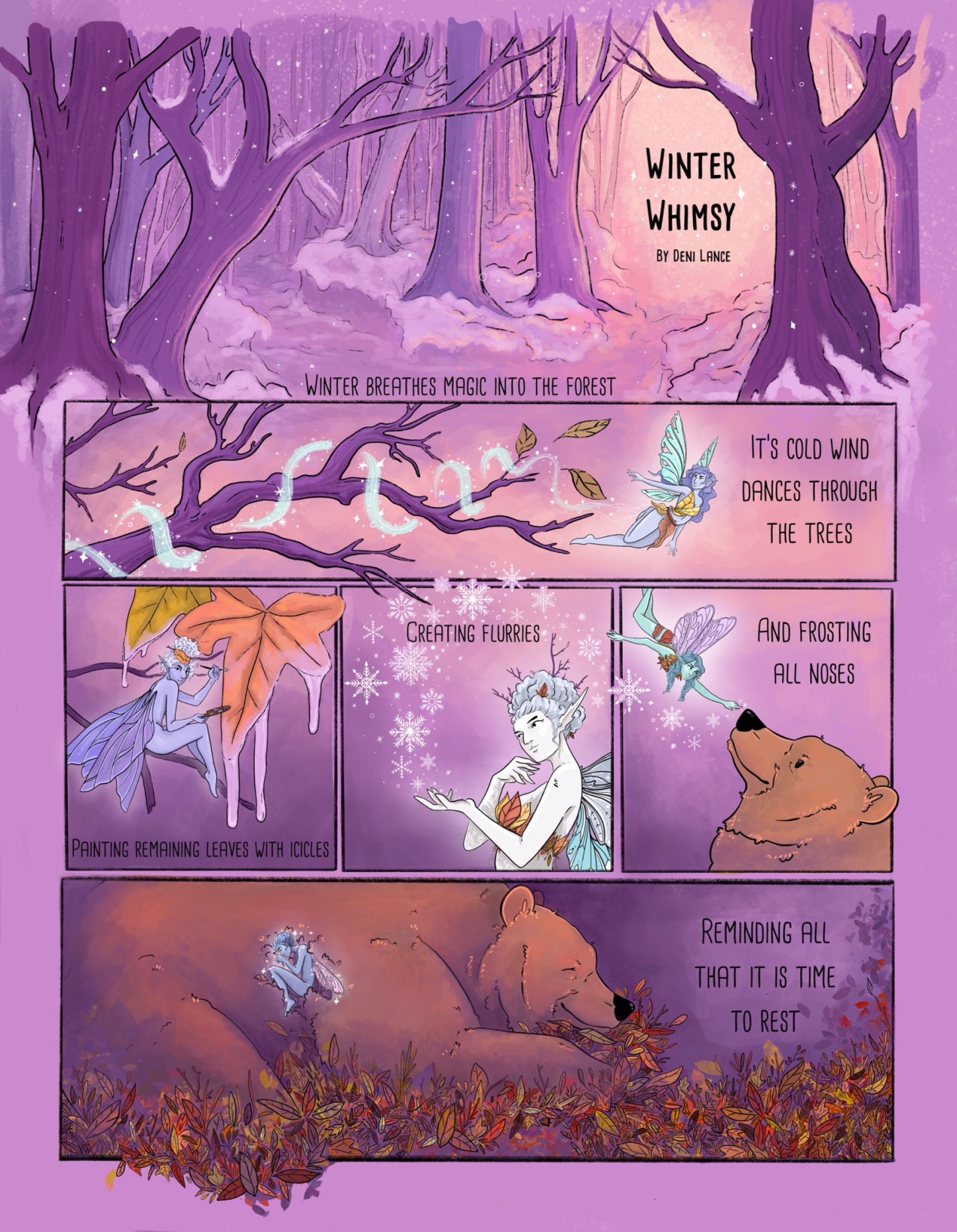The comic strip, titled "Winter Whimsy by Denny Lance," features a vibrant winter forest scene with a background of purple and pink hues. At the top, a misty aura surrounds purple trees bordered by snow, framing the title. Below, an enchanting narrative unfolds with the subtitle, "Winter Breeze Magic Into the Forest."

In the first panel, a long rectangular frame, a purple branch stretches outward, enveloped in a blue and white magic aura with three fluttering leaves. A fairy with cyan wings, purple hair, an orange-yellow shirt, and a brown leg covering, their grayish-blue skin glowing, creates the magical scene. To the right, the text reads, "It's Cold Wind Dances Through the Trees."

Moving to the left, another fairy with purple wings, short curly white hair, and similar skin, sits on a small brown branch adorned with large orange and green leaves, dripping with icicles. The inscription beneath this panel states, "Painting Remaining Leaves with Icicles."

The next close-up panel highlights this fairy, now featuring whiter skin and gray-cyan wings, holding three leaves of yellow, orange, and greenish-yellow hues. Her pointed ears and short grayish-blue hair, interspersed with small branches, are prominent. The magic snow flurries around her as the text reads, "Creating Flurries."

The narrative then shifts to a brown bear looking up at the fairy, who now has dark blue or green skin, blue hair, purple wings, a brown shirt, and red pants. "Enfrosting All Noses," reads the text, with snow flurries speckling the scene.

In the final panel, a vibrant bed of leaves in brown, red, green, and yellow mixes together, creating a cozy atmosphere. The fairy sleeps atop the bear, and the text on the right reads, "Reminding All that it is Time to Rest." This whimsical tale captures the serene magic of winter as it breathes life into the forest.